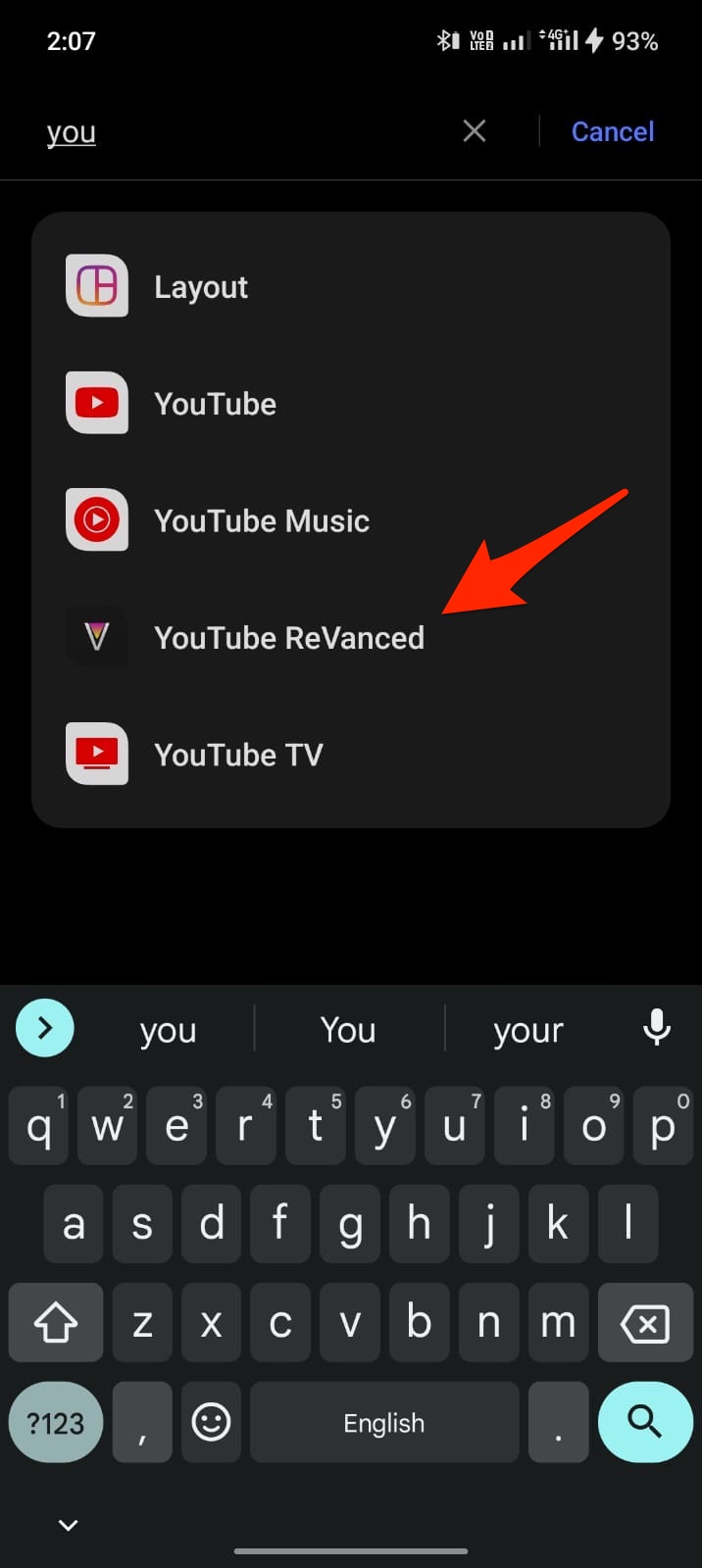The image is a mobile screenshot from a website displayed on a phone. The background is black, and at the very top of the screen, the time reads 2:07, though it does not indicate whether it is a.m. or p.m. On the upper right side, the battery icon shows a charge level of 93%. 

In the center of the image, there is a dark gray box, offering a slight contrast against the black background. Within this box, several YouTube-related icons are listed from top to bottom. In white font, the first entry is "YouTube," accompanied by the familiar YouTube logo: a red square with rounded edges and a white triangle pointing to the right. Below this is "YouTube Music," which features a similar logo but in a circular shape. The third entry is "YouTube ReVanced," represented by a stylized letter "V." Finally, at the bottom is "YouTube TV," where the logo resembles a red square that symbolically depicts a TV set or flat-screen television. 

At the very bottom of the screenshot, the virtual keyboard is visible. The keyboard's background is very dark gray, with the keys being a slightly lighter shade of gray and the letters in white font.